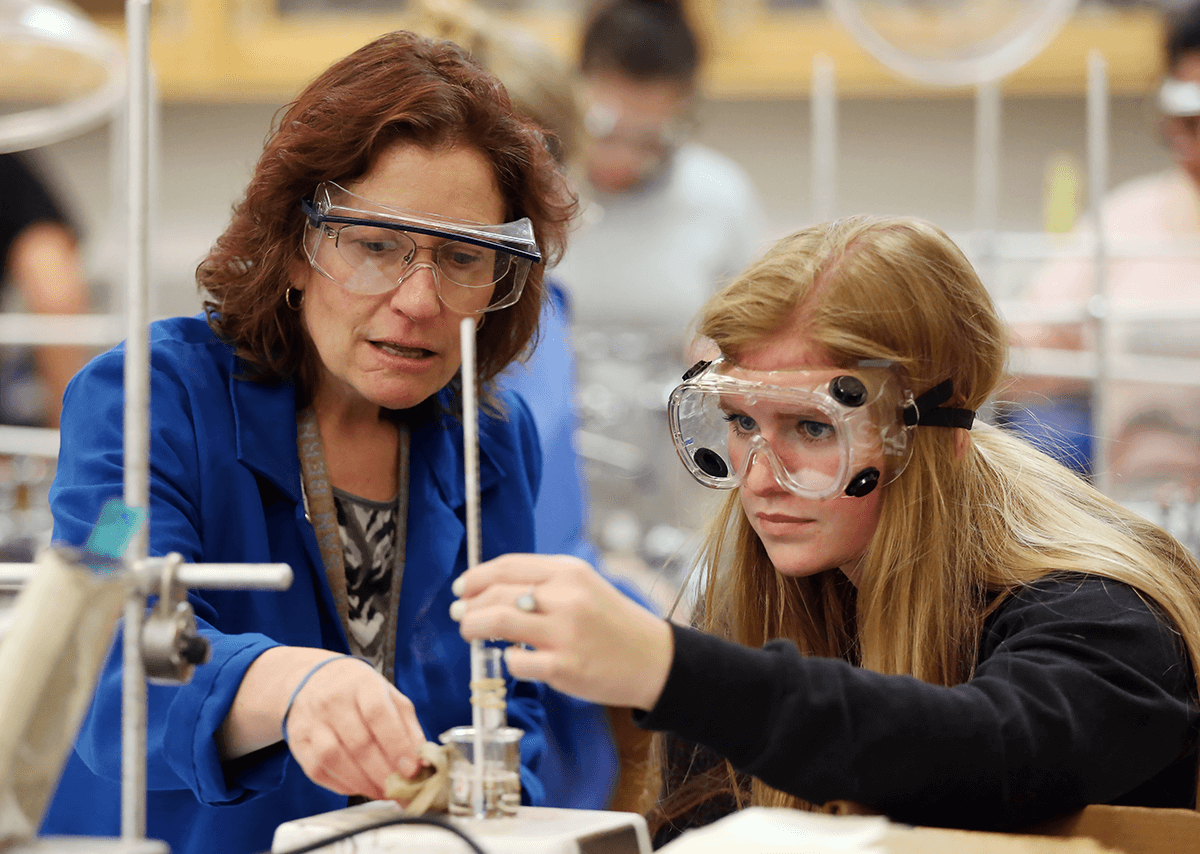In this detailed color photograph, two women, likely engaged in a scientific experiment, are prominently featured. The older woman on the left, who appears to be the teacher, is wearing safety goggles over her eyeglasses, a blue jacket over a black and white shirt, and a blue bracelet on her right wrist. Her reddish-brown hair falls to her shoulders, and she has a lanyard around her neck. The younger woman on the right, who looks to be seated, has long, straight strawberry blonde hair and is dressed in a black long-sleeve shirt. She also wears safety goggles and has a ring on the third finger of her left hand. Both women are focused on a piece of scientific equipment on the table, possibly a tube filled with liquid, indicative of a science project or experiment. The background is blurry, revealing vertical bars and a lock in the lower left corner, giving the impression of a lab or classroom setting. Another individual wearing safety goggles can be faintly seen in the background, further supporting the educational context of the scene.